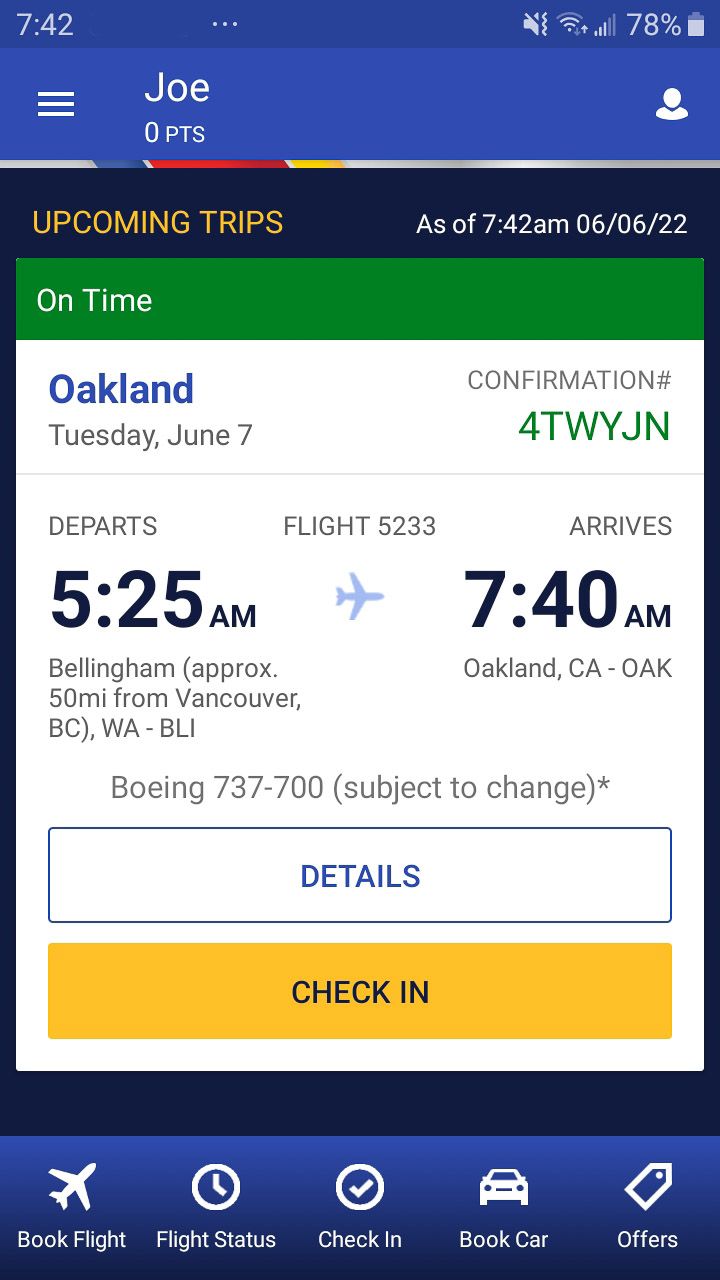**Caption:**

A screenshot of a mobile phone display with a vertical rectangular layout and a medium blue background. In the top left corner, the time is indicated as 7:42, while the battery level is shown as 78% in the upper right corner. Below this, three horizontal lines are followed by the name "Joe" in white font with "0 PTS" next to it.

The background transitions to a darker blue where "UPCOMING TRIPS" is displayed in bold, yellow, all-capital letters on the left side. To the right, in white font, it states "as of 7:42 AM, 06/06/22."

A green rectangular section beneath this says "ON TIME" in white font. The next section features a white background. In the top left corner, "Oakland" is written in blue font. On the opposite side, "CONFIRMATION" is in black, all-capital letters. Below "Oakland," the date "Tuesday, June 7th" is mentioned. The confirmation code "T-W-Y-J-N" is in green under "CONFIRMATION."

Further details include "DEPARTS" in black, all-capital font, with a large, bold "5:25 AM" beneath it. Next to "DEPARTS," it says "Flight 5233" in light black font, then "ARRIVES," followed by "7:40 AM" in bold font. Beneath this arrival time, there's "Oakland, California - OAK." Below "5:25 AM," there's "Bellingham (approximately 50 MI from Vancouver, BC) - WA-BLI." Then it lists "Boeing 737-700, subject to change."

A white horizontal rectangular area with a blue border displays "DETAILS" in the center in blue, all-capital letters. Below this section is another similar bar in yellow with blue lettering that says "CHECK-IN." Across the bottom, a blue horizontal section contains options in white font with icons above: "Book Flight," "Flight Status," "Check-In," "Book Car," and "Offers."